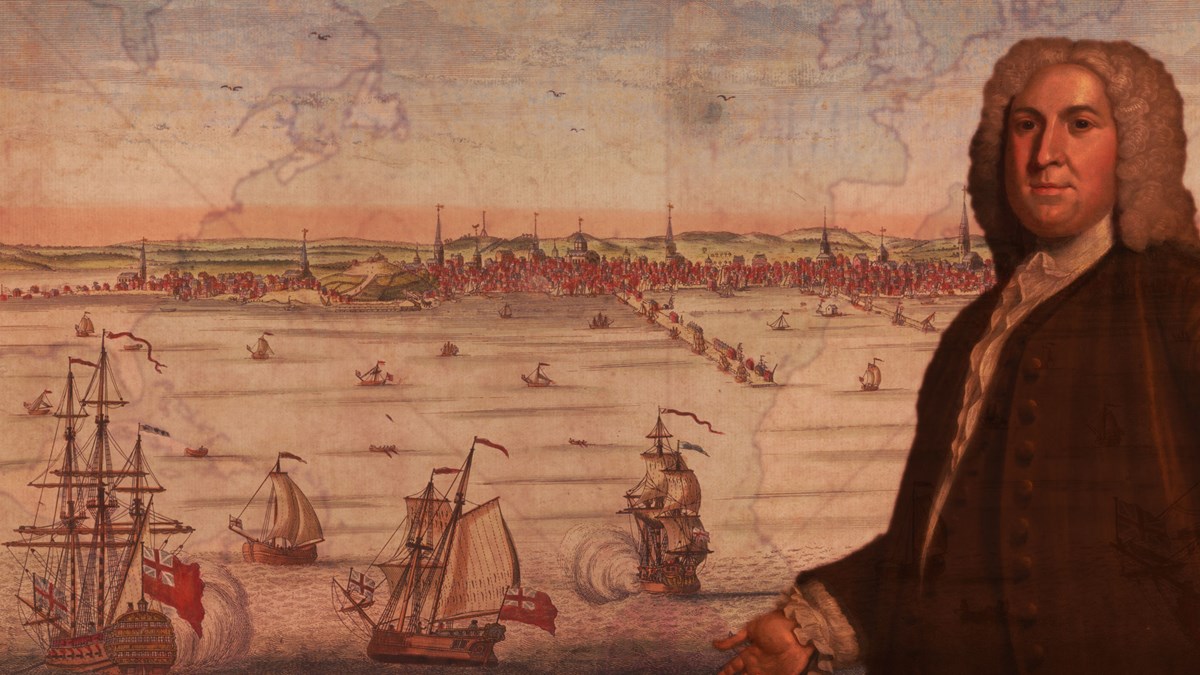In this detailed painting, set against a muted backdrop of vintage golds, ambers, light greens, and beiges, we find a prominent image of a historical figure on the right-hand side. The man, clearly from the 16th to 18th century, is depicted with a distinctive white powdered wig and dressed in an elaborate dark coat and a white ruffled shirt, reminiscent of the founding fathers of America. The background of the painting features a sky that transitions into a landscape composed of rolling hills, a town with red-roofed buildings, and church spires. In the left section of the artwork, several grand old-time sailing ships, adorned with likely British flags, traverse pale, almost-muted white waters, seemingly heading towards the west side of the painting. An intriguing element is a faint map superimposed over the entire image, with blurry yet recognizable outlines that resemble the geography of Europe or possibly Alaska, adding a layer of historical mystery and exploration to the piece.